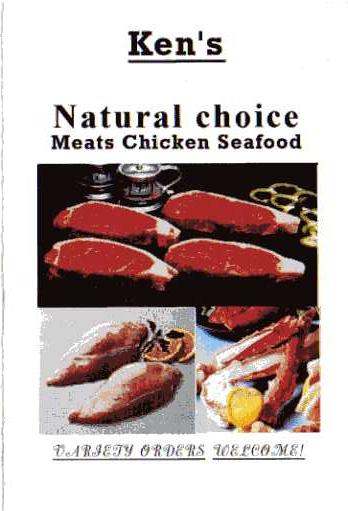The advertisement for Ken's Natural Choice Meats, Chicken, and Seafood features a clean white background with a prominent black line running vertically along the left side. At the top-center, "Ken's" is bolded and underlined in black text, followed by "Natural Choice Meats, Chicken, Seafood" written underneath. The ad showcases three distinct color photographs in a portrait orientation. 

The largest photograph at the top displays four raw steaks with white fat at the edges, suggesting they are ready to be cooked. Behind the steaks, there's a tin, which looks like a muffin tin, and a cup. Below this, on the left, there is a smaller photo of two chicken breasts garnished with orange slices. To the right of this, another small photograph depicts crab legs garnished with lemon slices. 

The ad concludes with the text "Variety Orders Welcome!" in fancy cursive script at the bottom. The style merges photographic realism with graphic design typography, creating a compelling and detailed visual appeal for Ken's meat and seafood offerings.